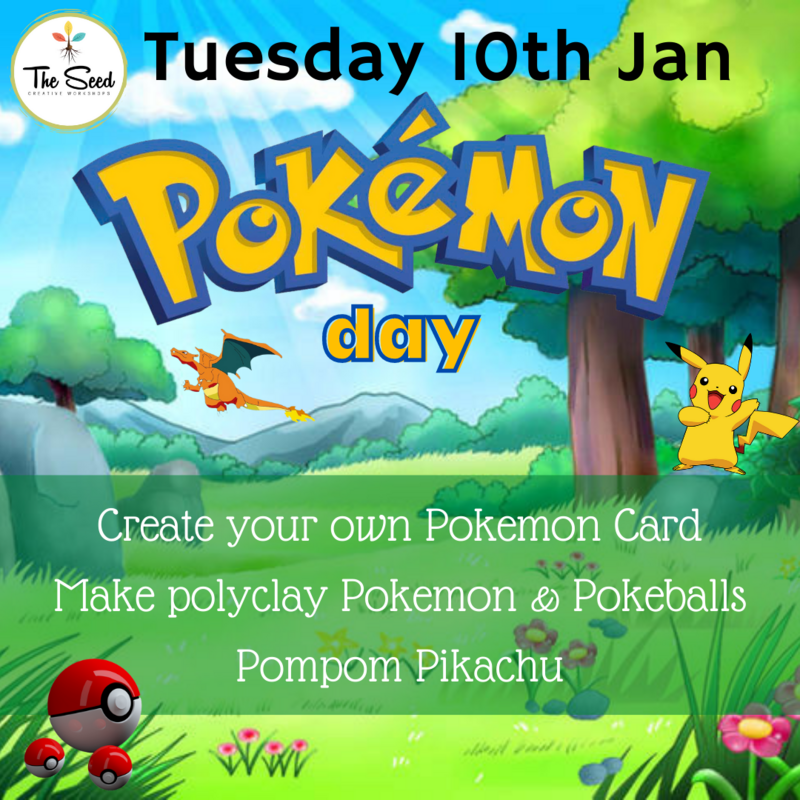A vivid landscape stretches out under a clear blue sky dotted with fluffy clouds. The foreground features a lush grassy field interspersed with large boulders on both the left and right sides. The scene is framed by trees on either side, with purple flowers adding bursts of color to the greenery. In the distance, majestic mountains provide a stunning backdrop. 

Dominating the upper left corner of the image is a circular logo with tree roots intertwining around it. The word "Seed" is inscribed inside the circle, and next to it, the text "Tooth Day 10th January" is printed. Below the text, the iconic yellow Pokémon logo, outlined in blue, is prominently displayed. 

Adding to the fantastical elements of the scene, an orange dragon soars gracefully near a tree while a Pikachu, perched atop a rock, captures the viewer's attention. The image is bordered with text that encourages creativity: "Create your own Pokémon cards, make polyclay Pokémon, and Pokémon pom-pom Pikachu."